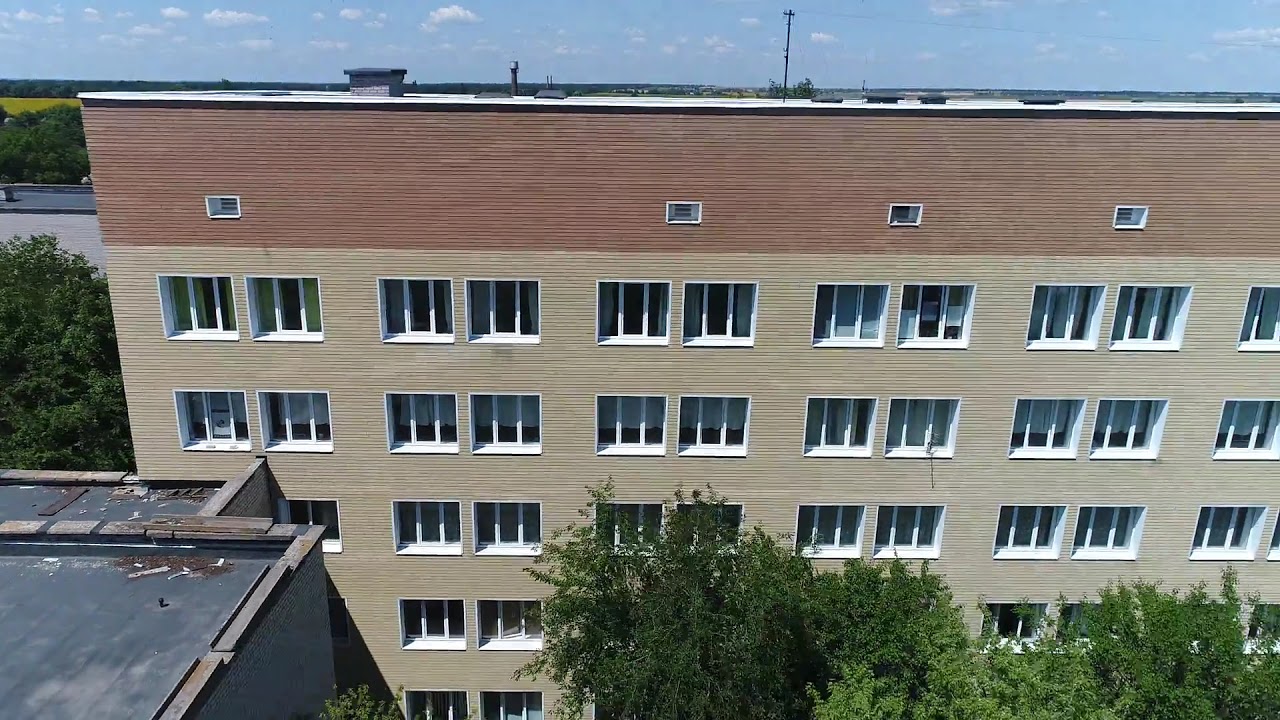The image features a multi-story, rectangular building prominently occupying the majority of the frame. The structure is composed of a mix of tan and reddish brick, with the reddish section located at the top of the building, housing smaller windows. The rest of the building showcases larger, three-panel windows framed in white, arranged in pairs that repeat consistently across five visible stories.

The scene also includes a tree with green leaves partially obscuring the view of the building from the front. On the bottom left, another rectangular building with gray siding and a black roof is visible. Surrounding the main structure, a gray parking lot extends to the left and is bordered by a lush green field with additional trees. Overhead, the sky is light blue with sparse clouds occupying the uppermost part of the image. The building features a white and black top section crowned with a central antenna, further adding to the detailed complexity of the scene.